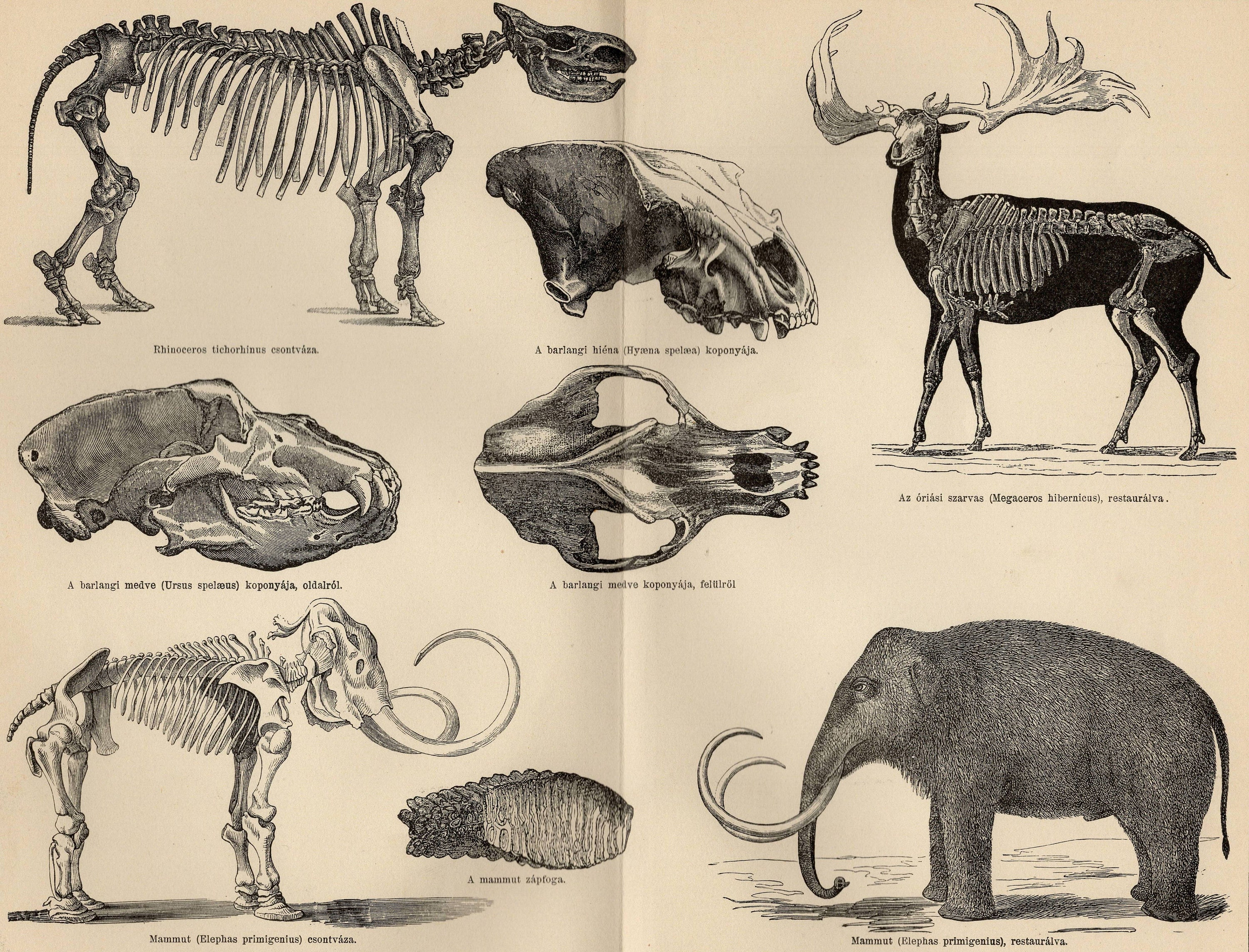The image displays a detailed spread from what appears to be a zoology or natural history book, showcasing various animal illustrations. The upper section features a moose with its notably large antlers, and the lower section highlights a woolly mammoth, distinguished by its long, curled tusks and trunk. The animals are depicted both in their external forms and as skeletons, illustrating their anatomical structure. Close-ups of their skulls are also included to allow for detailed comparison. Overall, there are eight distinct illustrations on the two pages, each accompanied by scientific names and unreadable labels. The background evokes the look of an old book with beige pages, giving the entire spread a vintage feel. The monochrome illustrations emphasize the evolutionary aspects and skeletal makeups of these deer-like and elephant-like creatures, providing a comprehensive overview of their physical characteristics.